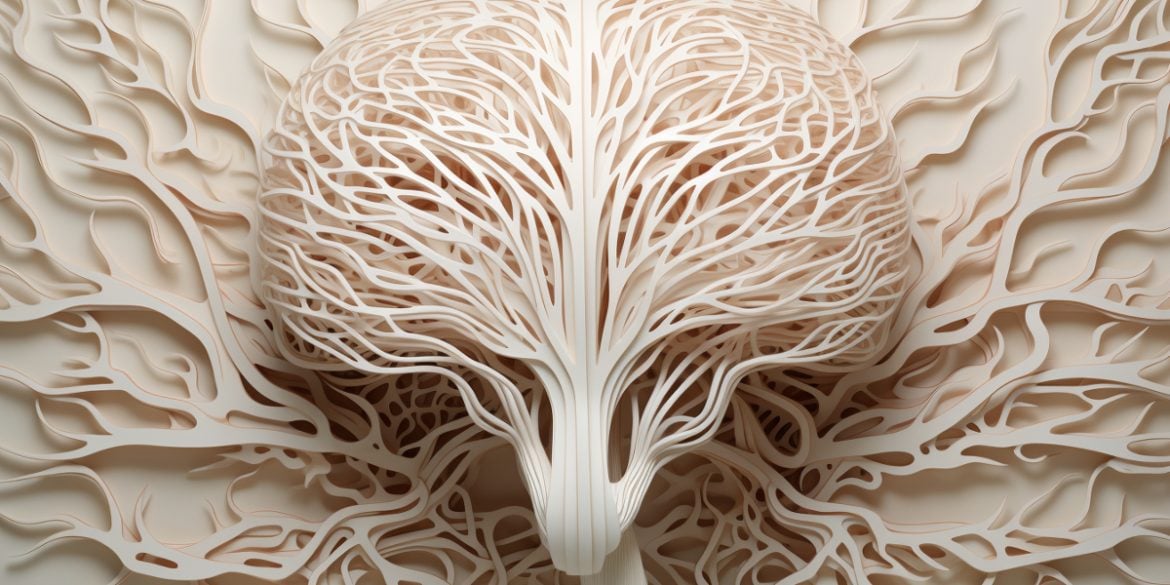The image portrays an intricate, abstract 3D model that appears to be etched or carved into a light-colored material, possibly wood or resin. The central figure vaguely resembles the general shape of a brain with its two hemispheres, though not anatomically accurate. It features numerous squiggly, interconnected lines that form this brain-like structure, offering a filigree quality with many openings through which light can pass. These lines are reminiscent of veins or flames and extend into the background, which also consists of similarly flowing, interconnected patterns. The entire scene might evoke associations with natural forms such as a mushroom, a celery stalk, or even exotic sea life anchored to an ocean floor, suggesting a blend of organic inspiration and artistic abstraction. The model may have been created using advanced 3D printing or carving machinery.